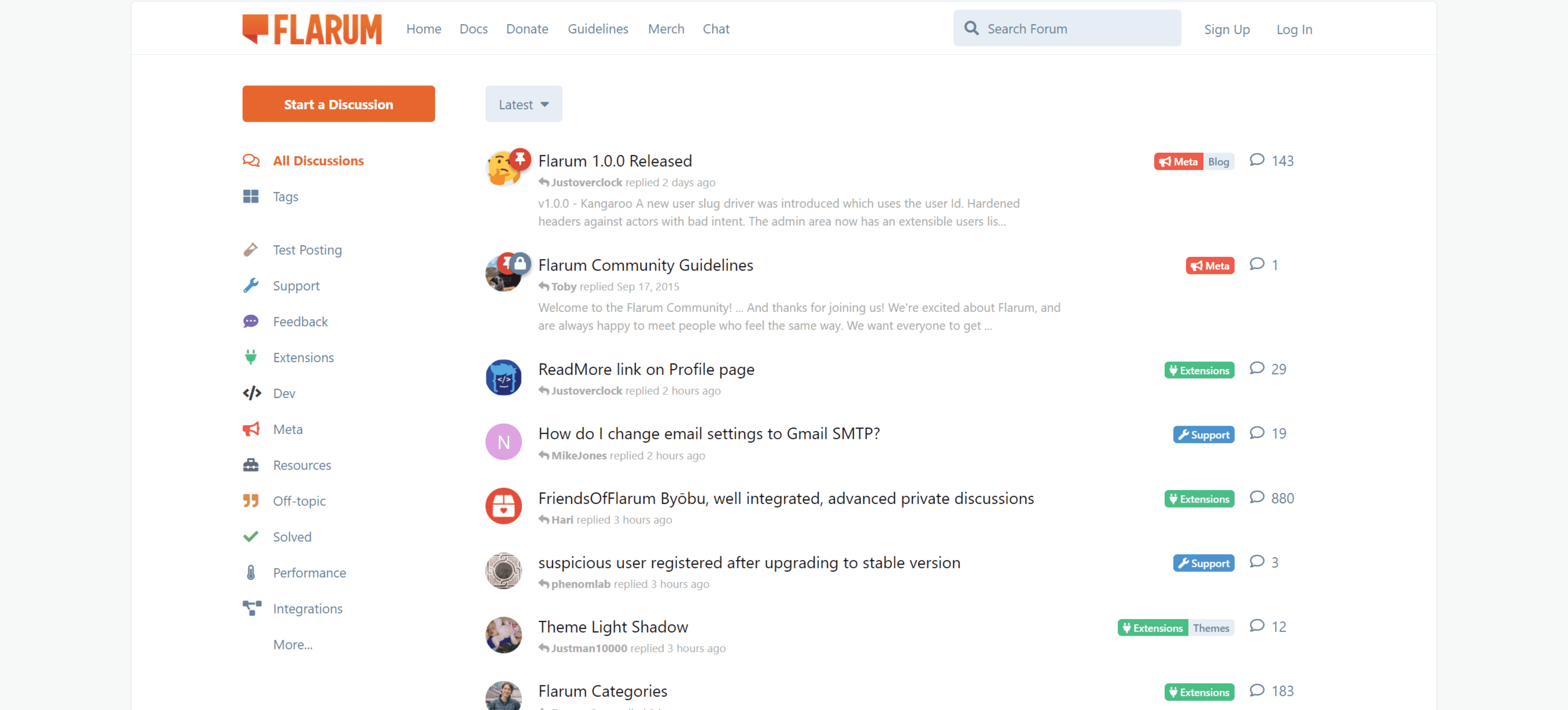This image is a comprehensive screenshot of a forum interface for a platform called FLARUM. The FLARUM logo, depicted as a rectangular chat bubble, appears alongside the platform's name in all-capitalized, elongated vertical orange letters. 

At the top navigation bar, several links are visible: Home, Docs, Donate, Guidelines, Merch, and Chat, with a search forum bar positioned to the right. Adjacent to the search bar, there are buttons for signing up and logging in. On the left side of the interface, there's a prominent large orange button labeled "Start a Discussion."

Beneath the main navigation, various tabs act as categories for the forum’s discussions, with "All Discussions" currently selected. Below these tabs is an option to add tags, followed by a list of existing tags including Text Posting, Support, Feedback, Extensions, Dev, Meta, Resources, Off Topic, Solved, Performance, and Integrations.

The central area of the screenshot displays the latest topics being discussed in the forum. Some visible discussion topics include:
- FLARUM 1.0.0 Released
- FLARUM Community Guidelines
- Read More
- Link on Profile Page
- How do I change email settings to Gmail, SMTP?
- Friends of FLARUM
- Vimeo
- Beoboo
- Well-Integrated Advanced Private Discussions
- Suspicious User Registered After Upgrading to Stable Version
- Theme Light Shadow
- FLARUM Categories

The visibility of these topics suggests that this forum serves a supportive role for the FLARUM community, focusing on issues and updates related to the platform.